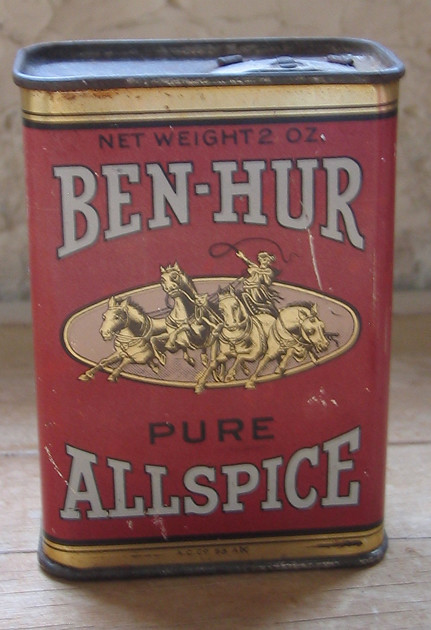This portrait-style image showcases an old, weathered, and slightly rusty rectangular cylindrical metal container of allspice, which exudes a vintage charm. The container, resting on a light-colored, whitish wood panel, features a predominantly red label. At the top of the label, in black text, it reads "Net Weight, 2 Ounces," followed by the brand name "Ben Hur" in bold white font. Central to the label is an illustration of a man riding a chariot drawn by four yellow horses, with a whip held high in the air. Beneath this image, the word "Pure" is printed in black, while "Allspice" appears at the bottom in white text. The can, despite its age and rust, still retains some of its gold edging at the top, where a tab for opening can be seen. The background suggests the setting is likely a kitchen, with a simple, brownish-gray wall.